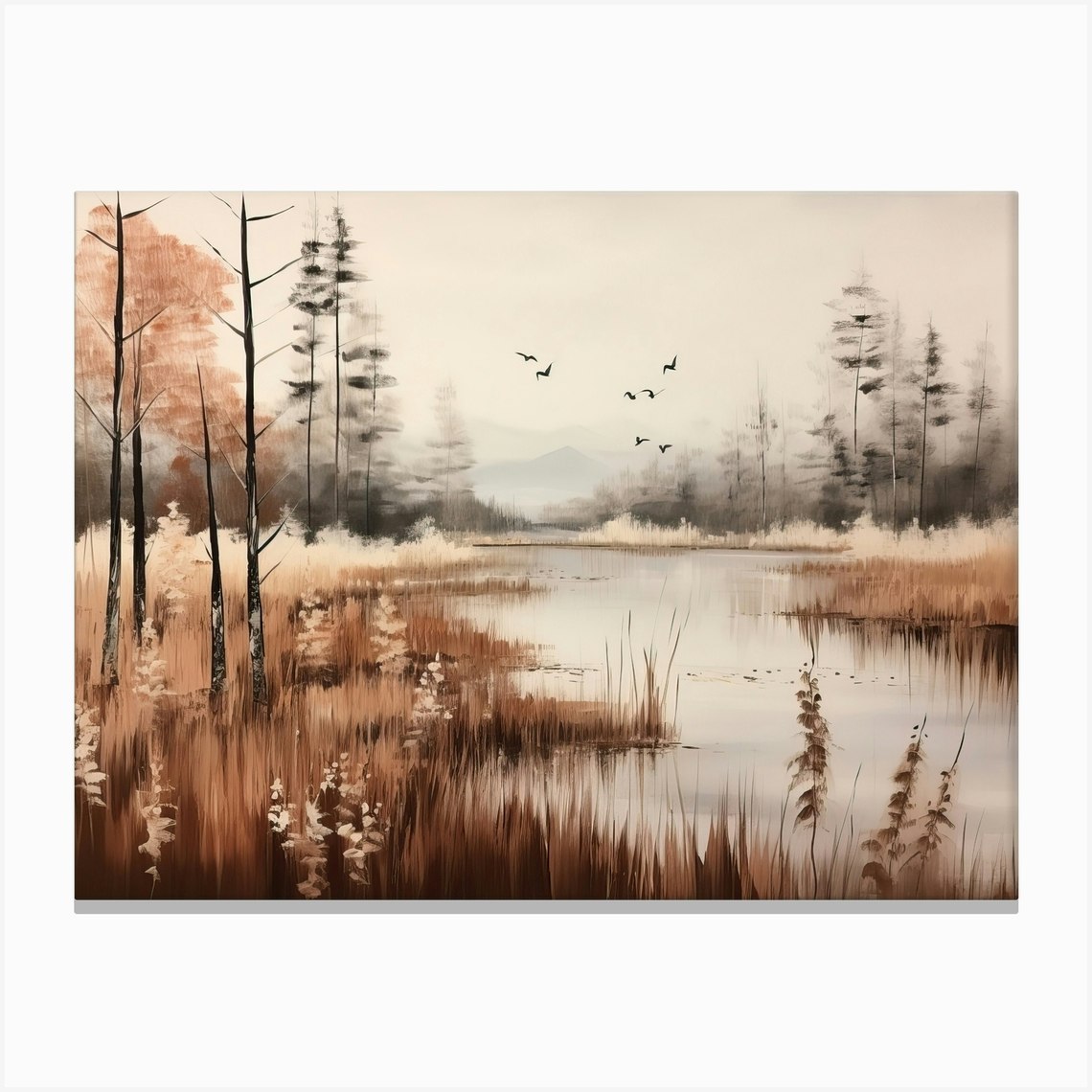This painting portrays a somber autumn landscape featuring a lake or swamp surrounded by barren and spindly trees, which can be seen prominently on both sides of the water. The sky is gray and misty, reinforcing the gloomy and overcast atmosphere of the scene. Tall grasses and reeds encroach into the murky water, mingling with various brown foliage and some white flowering plants or dying flowers that notably pop against the earthy tones. Birds can be observed in flight, receding into the distance and adding a sense of depth to the composition. In the far background, the tree shapes begin to fade into mist, revealing the faint outlines of mountains. The entire painting is rendered in a muted palette dominated by various shades of brown, beige, black, and gray, giving it a monochromatic and melancholic feel. The trees in the foreground are meticulously detailed, capturing the texture and appearance of their bark.